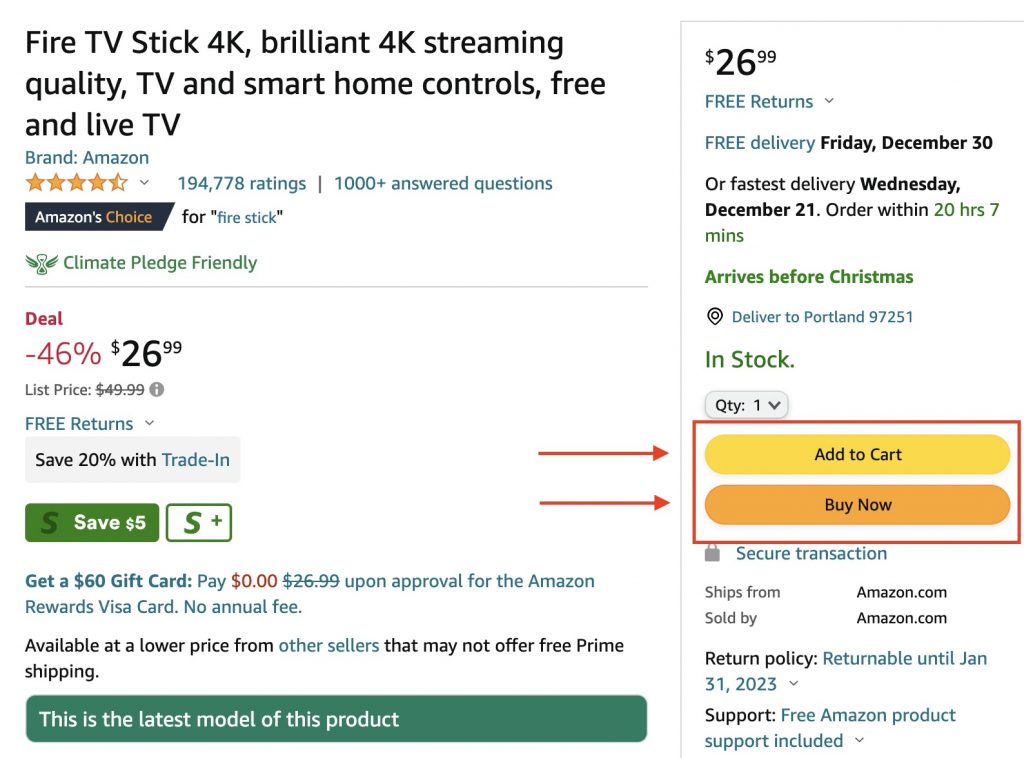**Caption:**

This is a screenshot from the Amazon website showcasing the Fire TV Stick 4K. At the top left, the product title is prominently displayed in bold black text, stating: "Fire TV Stick 4K - Brilliant 4K Streaming Quality, TV and Smart Home Controls, Free and Live TV." Below that, in blue text, is the brand name, Amazon. The product has a near-perfect rating, with 4.5 out of 5 stars filled in gold, based on 194,778 ratings. Additionally, there are over 1,000 answered questions, also highlighted in blue. The product is labeled "Amazon's Choice" for Fire Stick and is noted as "Climate Pledge Friendly" in green.

Beneath these details, there is a red highlight indicating a limited-time deal where the price is 46% off, bringing it down to $26.99 from the original $49.99 (the latter price being struck through). The offer includes free returns and mentions a 20% trade-in discount in a gray bar. Furthermore, there's a green bar offering an additional $5 savings with a clickable option. Customers can also apply for the Amazon Rewards Visa Card to receive a $60 gift card and have their annual fee waived.

Below, it mentions that the same product is available at a lower price from other sellers, which may or may not include free Prime shipping. This is noted as the latest model of the product. On the right-hand side, there are two prominent red buttons for "Add to Cart" and "Buy Now". The estimated delivery date, if ordered, is listed as free delivery by Friday, December 30th.